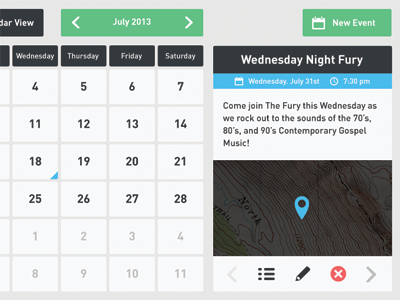In this image, we see a detailed view of a segment of a calendar. The top of the image features a light gray background with various categories. On the left corner, "DAR View" is displayed in white text on a black background. To the right, two categories have green backgrounds. At the center, the text "July 2013" allows for adjusting the calendar date, and next to it on the right, "New Event" is displayed in white text alongside a calendar icon.

Beneath these categories, the days of the week are listed horizontally: Wednesday, Thursday, Friday, and Saturday. The corresponding dates listed in black text are: 4, 5, 6, 7, 11, 12, 13, 14, 18, 19, 20, 21, and 25, 26, 27, 28. Below these, additional numbers in gray are displayed with white squares around them: 1, 2, 3, 4, and 8, 9, 10, 11.

On the right, there's a highlighted black background with the text "Wednesday Night Fury." Below that, a blue background notes an event on "Wednesday, July 31st, 7:30 PM," inviting attendees to "Come join the fury this Wednesday as we rock out to the sounds of 70s, 80s, and 90s contemporary gospel music" in black text on a white background.

At the bottom of the image is a partial map, showing a blue icon indicating a location, and a light gray background with several other icons surrounding the entire scene.